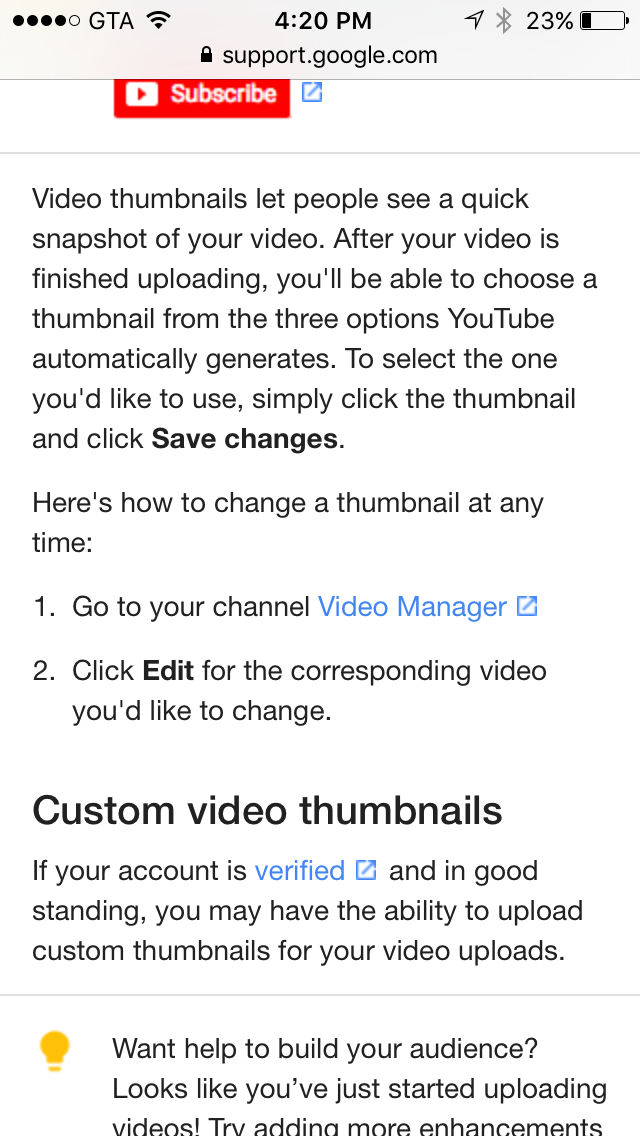This image is a detailed screenshot taken from a smartphone, capturing a Google support page about customizing video thumbnails. At the top of the screen, the status bar displays several icons: a series of dots followed by "GTA" indicating the location, a tornado symbol representing full Wi-Fi signal, the time reading 4:20, an arrow showing active location services, a Bluetooth icon, and a battery percentage at 23%. Below this, a lock symbol is visible, next to the URL "support.google.com".

The screenshot specifically shows a section of a Google support page with a red rectangular box at the top featuring a play button and the word "subscribe." Underneath, there's a detailed print description discussing video thumbnails and how to change them. Prominently, there's bolded text that reads "Custom video thumbnails," explaining the need for account verification to upload custom thumbnails for video uploads. Additionally, the terms "video manager" and "verified" are in blue and hyperlinked, suggesting these can be clicked to navigate to further information.

At the bottom of the screenshot, a yellow light bulb icon is visible, followed by tips on building an audience and adding enhancements to videos, providing helpful advice for the user.